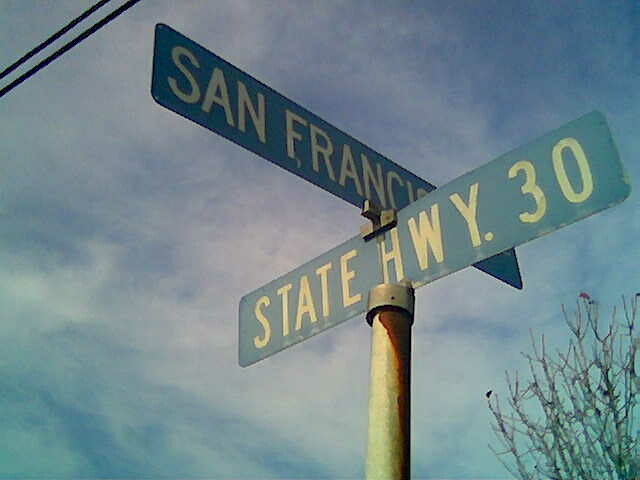This close-up photograph captures an upward view of two intersecting street signs mounted on a silver metal pole. The scene is set against a backdrop of a blue sky partially veiled by thin, sparse white clouds. Nude branches of a leafless tree stretch into view from the bottom right corner, while two power lines cut diagonally across the top left. The prominently displayed street signs are long and rectangular with a blue background and white text. The lower sign reads "State HWY 30" and the upper horizontal sign directs towards "San Francisco."